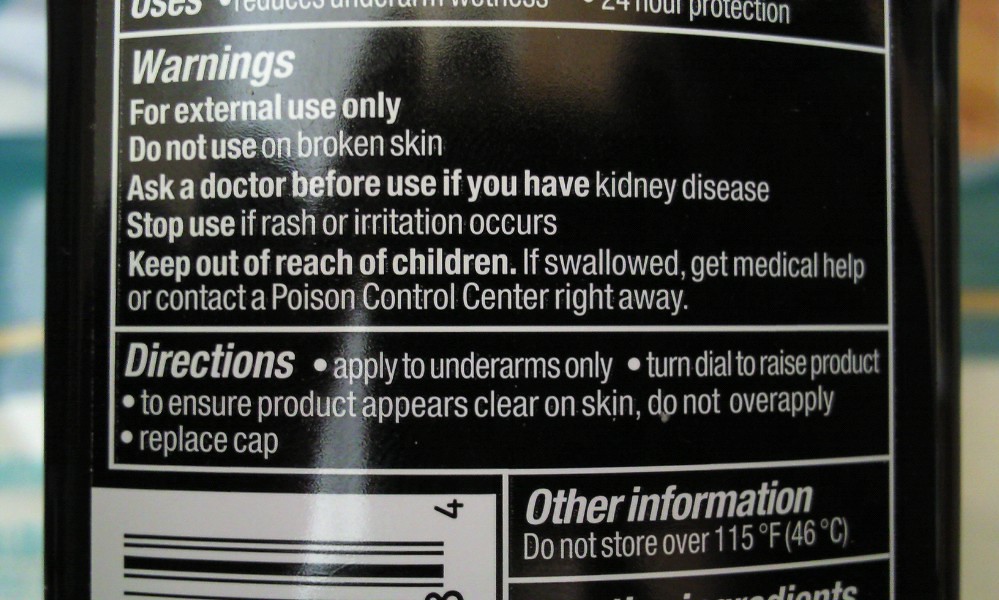This is a high-resolution photograph showcasing a black package adorned with sleek white font. The image quality is exceptionally clear, allowing for a detailed observation of the package's design and text. Positioned towards the bottom of the image is a partially visible barcode, hinting at the product's retail nature. The background features an artistic blur of colors, including shades of green, white, yellow, and a warm orangey tan, adding a visually appealing contrast to the primary subject.

The top part of the package label is partially visible, displaying the word "Uses," followed by informational text promoting "24 hour protection." Below this, a series of warnings advise: "For external use only," "Do not use on broken skin," and to consult a doctor before use if you have kidney disease. The text continues with important safety guidelines, such as stopping use if rash or irritation occurs, keeping the product out of reach of children, and seeking medical help or contacting a poison control center immediately if swallowed.

Further directions instruct to apply the product only to underarms, turn the dial to raise the product, and to ensure clear application by avoiding overuse. The information ends with practical advice on storing the product: "Do not store over 115 degrees Fahrenheit or 46 degrees Celsius."

This descriptive caption meticulously highlights both the visual and textual elements captured in the photograph, providing a comprehensive overview of the black package's appearance and informative label.